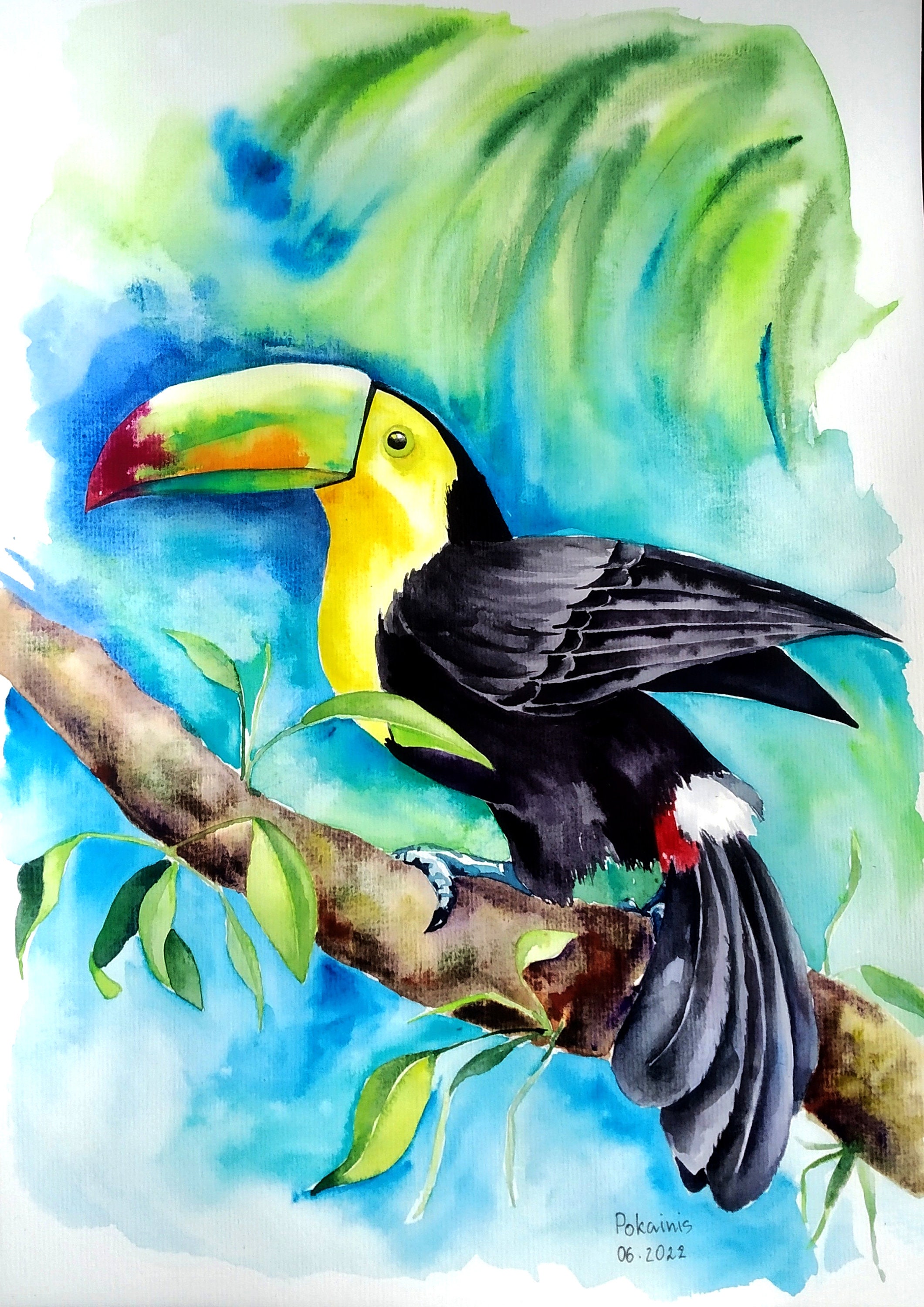This is a watercolor painting depicting a vibrant toucan in profile, facing towards the left. The toucan’s head and neck are a striking yellow, smoothly transitioning into a black body. Two distinct tufts of feathers adorn its tail, with the upper tuft being white and the lower tuft a vivid red. The bird's beak is predominantly green, accentuated with touches of orange and red near the tip. It is perched on a tree branch, displaying one visible claw with a leg that appears blue and talons that are black.

The background contrasts beautifully with the toucan, featuring a mix of lush green foliage and a sky colored in shades of blue, interspersed with swirls of white clouds. The sky and foliage are artistically rendered, with colors blending fluidly in a manner characteristic of watercolors. The image has a dynamic and whimsical feel, with the artist’s brushstrokes creating a sense of movement and vibrancy.

In the bottom right corner of the piece, the signature "POKANIS" is inscribed in black, alongside the date "06-20-22."